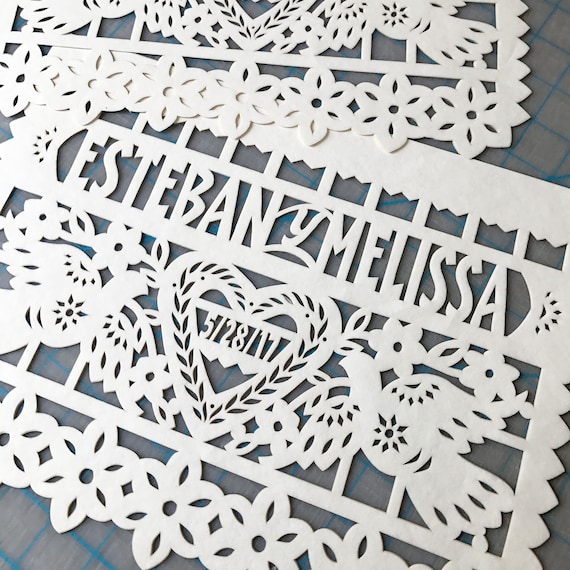This image showcases an intricately designed wedding invitation featuring delicate paper cut-out art. The upper portion is adorned with a solid white border that descends into pointed details, complemented by a series of fine white lines. In the center, the names "Esteban y Melissa" are prominently displayed, separated by a solid line beneath which lies an artistic arrangement of daisies and a heart. Central to the design is the heart, bearing the banner with the date "5-28-17" signifying May 28, 2017. Flanking the heart are two elegant white doves. The bottom edge of the card is accented with a floral border that spans its width. Interestingly, another card with a similar floral design at the bottom is overlapped at the top of the primary card, enhancing its layered effect and floral motif.